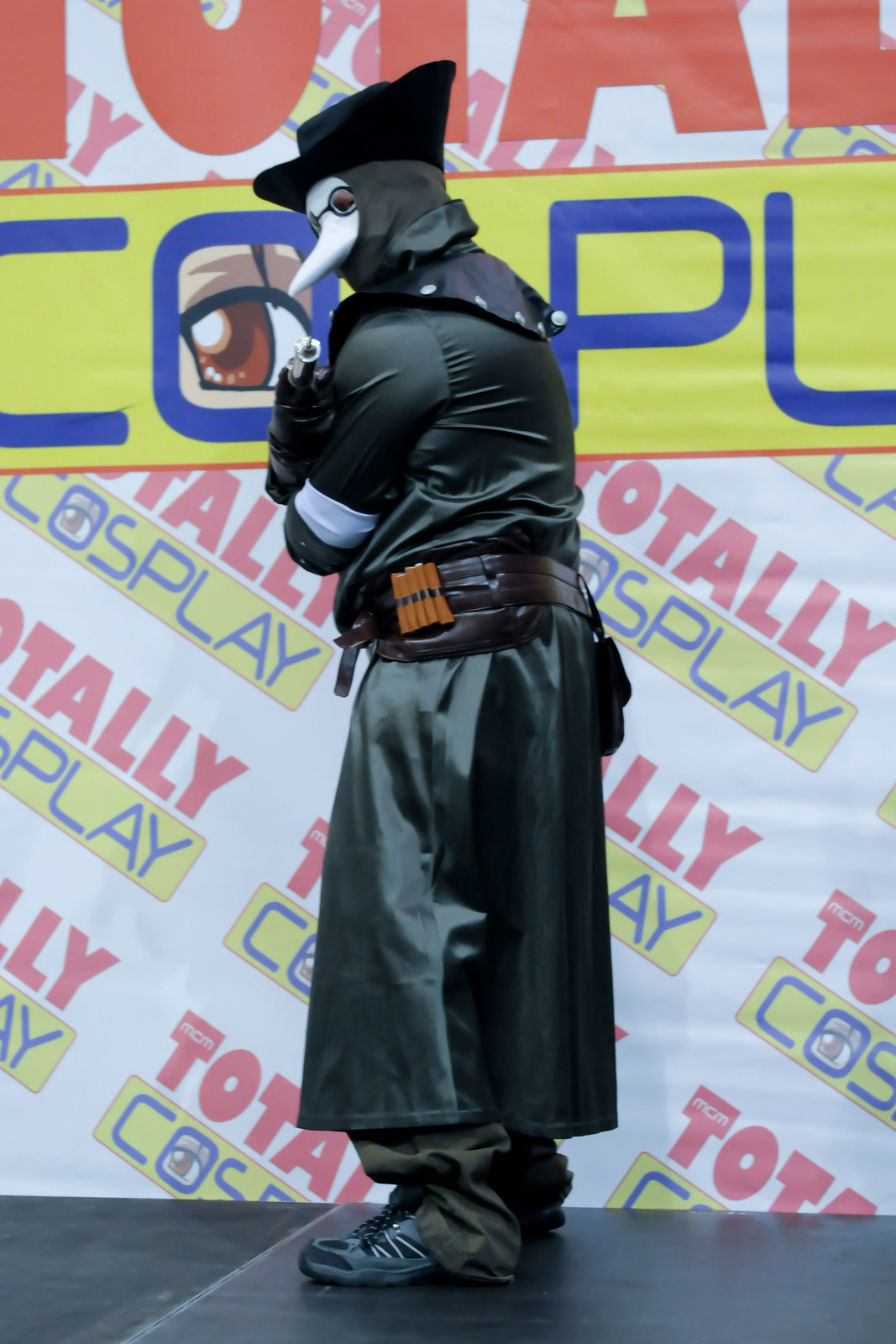In the photograph, a person is dressed as a historical plague doctor, standing in front of a backdrop that reads "Totally Cosplay" — with "Totally" in red, a yellow banner with blue text for "Cosplay," and an eye inside the 'O' of "Cosplay." The individual is facing to the left, giving us a clear profile view. Their outfit consists of a long, black raincoat or trench coat that appears to be leather-like, complemented by black shoes, black gloves, and a black hood. Over the hood, a black tri-cornered hat is perched, adding to the period costume's authenticity. A white armband is noticeable on their left arm, and a belt, which appears to contain cylindrical objects possibly resembling bullets or tubes, is strapped around their waist. The highlight of the attire is a white beaked mask with drawn-on round black glasses around the eye holes, characteristic of the plague doctors of old. The black ground they're standing on has a glossy, wet concrete appearance, enhancing the setting of this event. The person also holds an indistinct metallic object in their right hand, further contributing to the mysterious and historically themed costume.